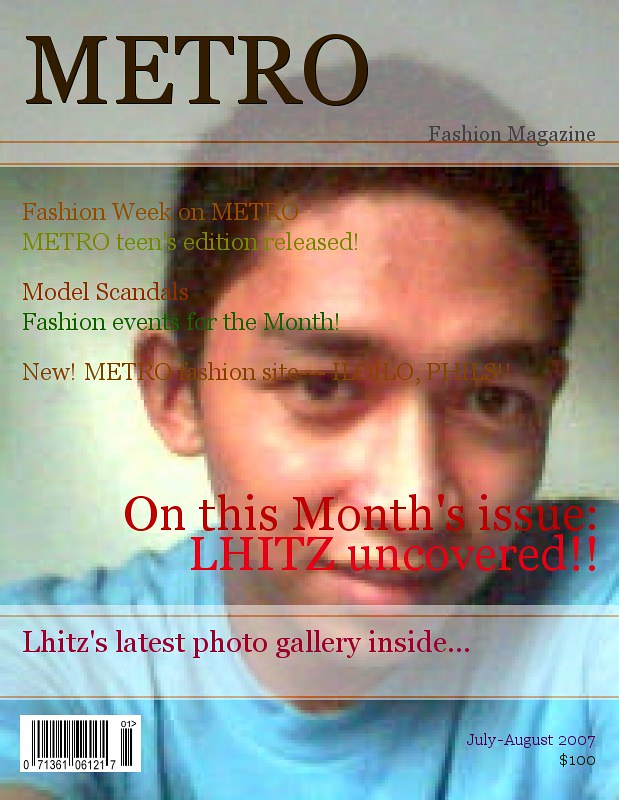The image depicts the front cover of Metro Fashion Magazine featuring a medium-dark-skinned young male with a mixed ethnicity appearance, likely a blend of Asian and Black. He has short dark brown hair, dark eyes, and dark eyebrows, and is clad in a short-sleeved turquoise shirt. Central to the cover, the title "METRO" is prominently displayed in big black capital letters at the top. Over the man's face, in bold red text, are the words "ON THIS MONTH'S ISSUE: LHITZ UNCOVERED! LHITZ'S LATEST PHOTO GALLERY INSIDE!" The left side is adorned with various texts: "Fashion Week on METRO" in orange, "METRO Teens Edition Released" in green, "Model Scandals" in red, "Fashion Events for the Month" in evergreen, and "New METRO Fashion Site" in orange. The entire backdrop of the cover is gray, with the text in varied vibrant colors. The bottom left corner features a barcode, while the bottom right hand corner denotes the date "July-August 2007" and the price "$100".